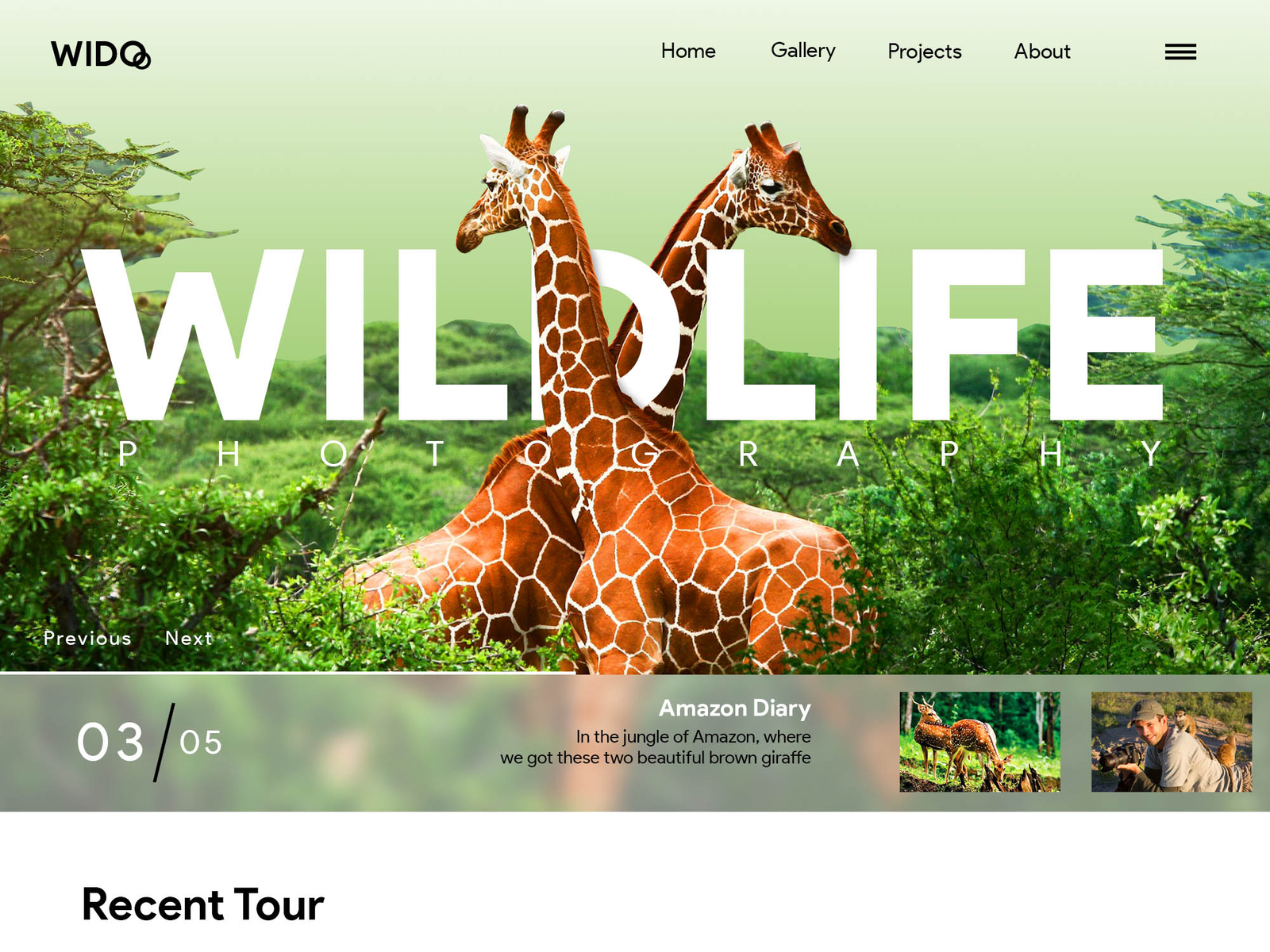This vibrant wildlife photography website features a central banner with the text "Wildlife Photography" in striking white font. In the top-left corner, the logo "WIDO" is prominently displayed. The top-right corner hosts navigation tabs labeled Home, Gallery, Projects, and About, along with a three-lined menu button for additional options.

At the bottom-left of the banner, the notation "03/05" indicates that visitors can browse through five different featured photos. In the bottom section of the page, titles such as "Amazon Diary" and "The Jungle of Amazon" introduce a stunning image of two brown giraffes, captured standing side by side but facing in opposite directions.

Complementary to the main image, two small thumbnails are positioned in the bottom-right corner, providing a preview of other notable photographs. This well-organized and visually appealing layout enhances the viewer's experience, seamlessly showcasing the beauty and diversity of wildlife photography.